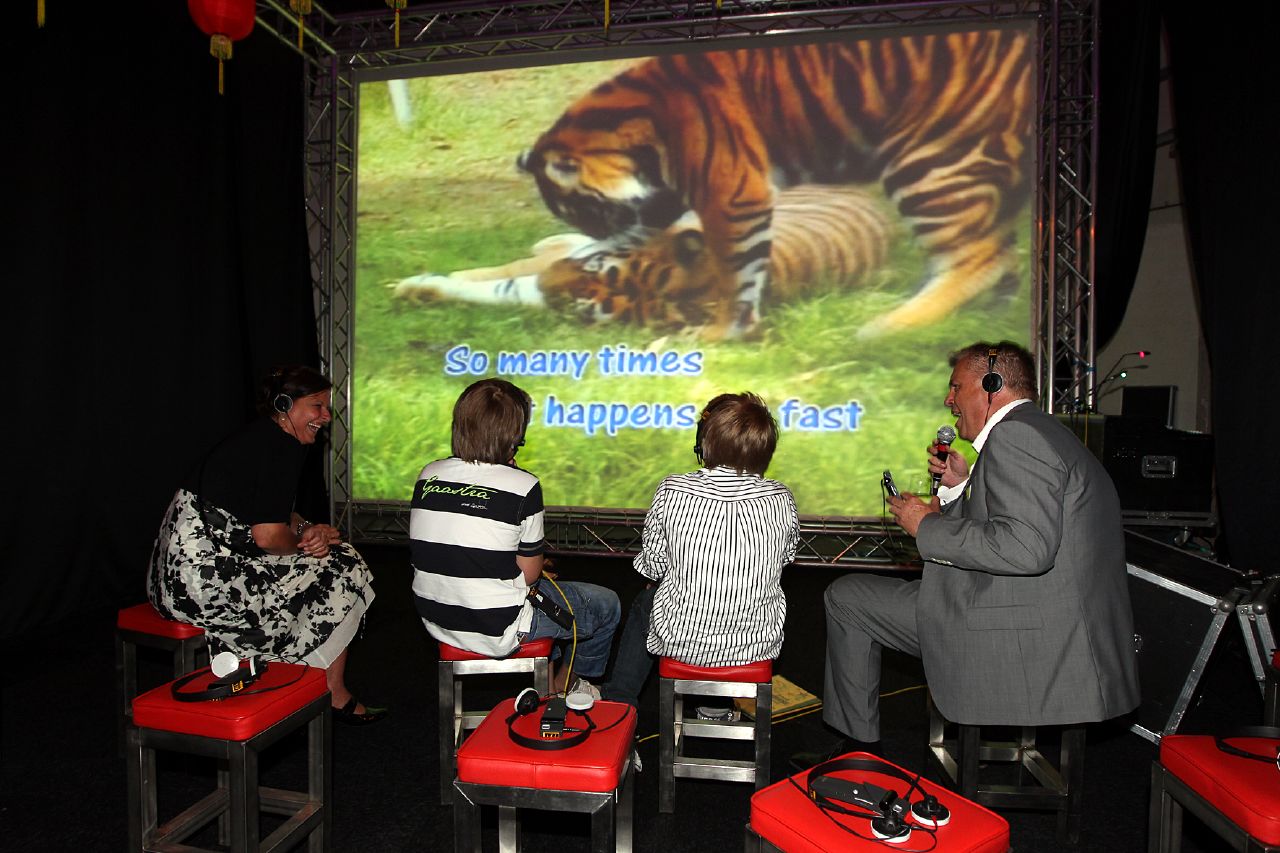This color photograph captures a scene from behind four individuals seated on small red benches, engrossed in watching a large screen. From left to right, the viewers include a middle-aged woman partially turned to the right, caught mid-laugh, followed by two young boys around 10 to 12 years old, both dressed in black and white striped shirts with light brown hair, their backs to the camera. On the far right sits a middle-aged man in a gray suit with a white dress shirt, holding a microphone and wearing headphones, slightly turned towards the others. The large screen they are facing displays two tigers, one standing over the other, amidst green grass, with the text "so many times it happens so fast." The setting appears to be indoors, featuring additional stools lined up behind them. The scene is bathed in a variety of colors including light blue, orange, white, gray, black, red, green, and silver, with elements like metal casings and frame structures visible around the screen area.